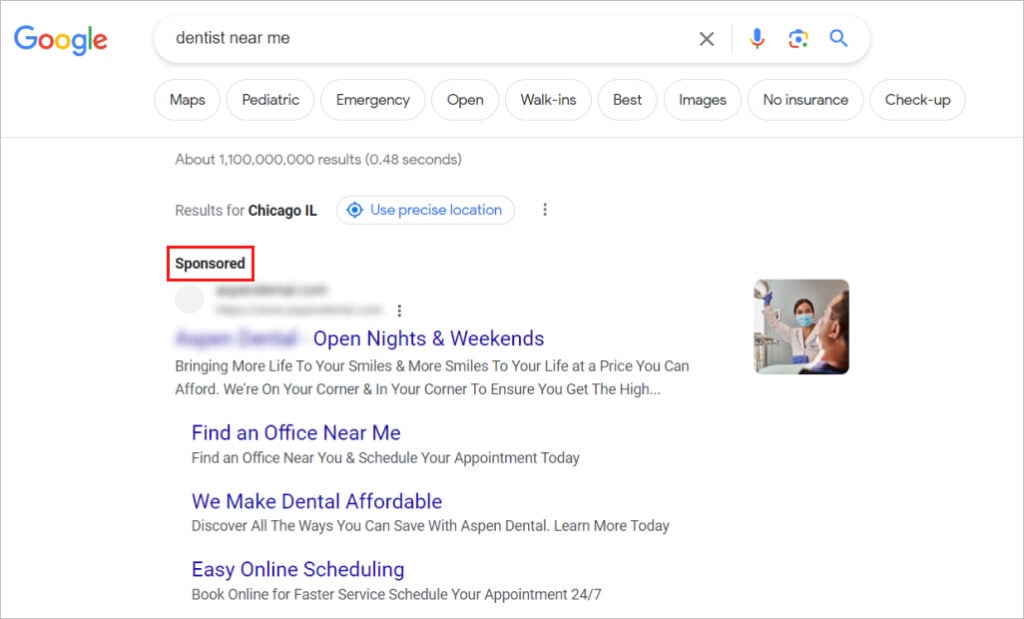This image captures a detailed view of a Google search page with a query about "dentists near me." 

The background is entirely white and features the familiar Google logo at the top center of the page. A thin black border surrounds the entire image. To the right of the Google logo is a large search bar containing the query "dentists near me" in black text, with an "X" on the far right for clearing the text. Adjacent to the search bar are icons: a blue search icon, a camera icon in red, yellow, and blue, and a voice search icon in blue.

Just below the main search bar, there is a row of tabs with white backgrounds and black text, labeled: "Maps," "Pediatric," "Emergency," "Open," "Walk-ins," "Vest," "Images," "No Insurance," and "Checkup." Beneath these tabs is a thin black line displaying search result details such as the number of results and the time taken to generate them. This line also specifies that the results are for Chicago, Illinois. 

To the right of the search details is an additional search bar with a white background and an icon resembling a scope or magnifying glass. Next to it in blue, it says "Use precise location." 

On the left side under the Chicago location information, there is a red-bordered area labeled "Sponsored" in white text and black letters. Below this section, three lines are blurred out, followed by a blue text that reads "Open nights and weekends" with accompanying lines of information.

Further down the page, slightly left-aligned, is text stating "We make dental affordable," "Easy online scheduling," with corresponding lines of information. To the right, the text repeats "Open nights and weekends" accompanied by an image of a nurse assisting a patient.